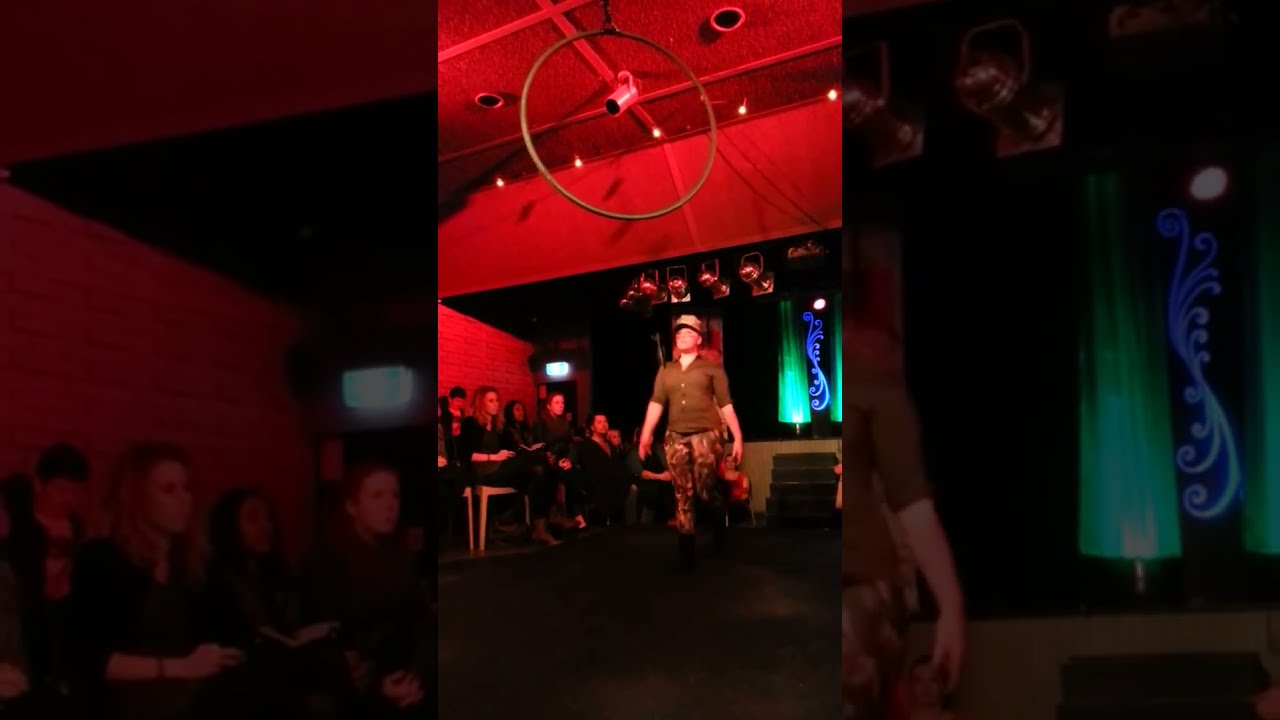In the image, a serious-looking woman stands at attention in the center of a bar, which is bathed in intense red light. She is wearing a very tight olive green long-sleeve polo shirt, camouflage pants tucked into boots, and a military-style baseball cap. Her outfit emphasizes a disciplined, almost militant appearance. Behind her, a variety of people are seated, some watching her attentively while others have their heads down. The bar, characterized by its vivid red lighting, has a ceiling adorned with five lit light bulbs and a thin black ring hanging above the woman. The surrounding architecture includes steps leading from what appears to be a stage area down to where she stands, and a structural metal grid supporting the lights. The scene is framed by large black rectangles on both the left and right sides, which run from the top to the bottom edges of the image. Mixed in the background is a subtle blend of teal and blue lights, contributing a swirl design and a slight contrast to the dominant red ambiance.